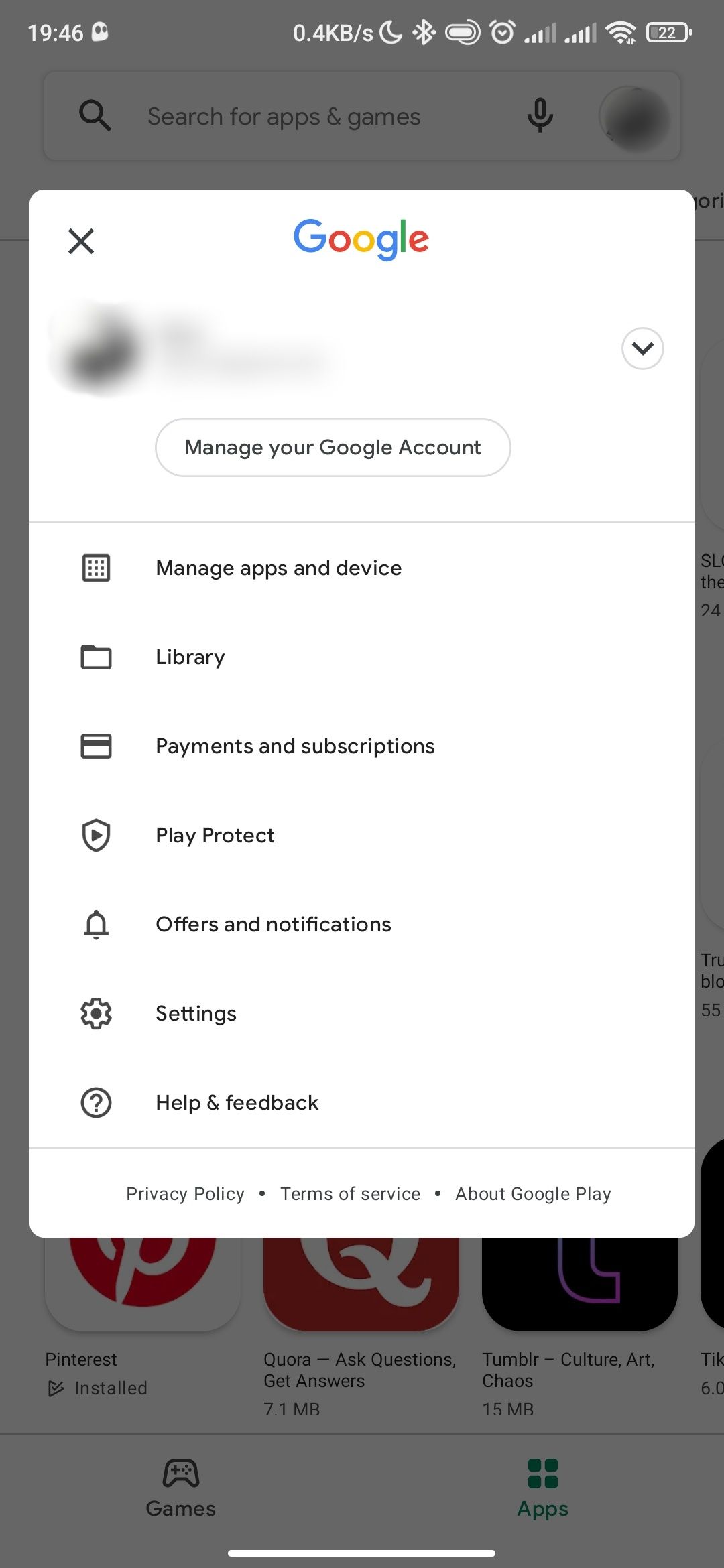The image features a smartphone screen with various details. At the top left corner of the screen, the time is displayed as "19:46" within a small white bubble. To the right, it shows "04KB/S" alongside several icons: a moon symbol, a Bluetooth icon, a white button, a stopwatch symbol, two network signal indicators, and a battery icon displaying a 22% charge.

Below this top bar is a white box with a black 'X' in the upper left corner. Central to this box is the word "Google" in multicolored letters. Underneath the Google logo is a call-to-action button labeled "Manage your Google Account" in black text. Following this is a thin grey line, under which there are several grouped icons with corresponding labels:

1. A box with dots labeled "Manage apps & device."
2. A folder icon labeled "Library."
3. A credit card icon labeled "Payments & subscriptions."
4. A shield with a triangle icon labeled "Play Protect."
5. A bell icon labeled "Offers & notifications."
6. A gear icon labeled "Settings."
7. A question mark in a circle labeled "Help & feedback."

At the bottom of the white box, after another thin grey line, there are links to "Privacy Policy," "Terms of Service," and "About Google Play." In the backdrop, a shadowed area is faintly visible, showing some app icons.